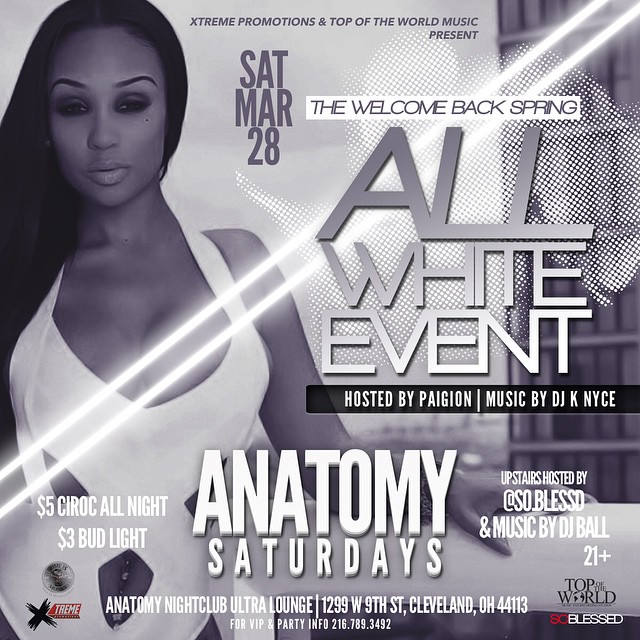This black-and-white poster advertises a musical dance event called the "Welcome Back Spring All-White Event," taking place on Saturday, March 28th. The event is hosted by Pagion with music provided by DJ KNYCE. At the top of the poster, "Extreme Promotions and Top of the World Music Present" is written in black. 

On the left side of the image is a photograph of an attractive young black woman with long hair, wearing a revealing white dress. Next to her, the poster highlights drink specials: "$5 Ciroc All Night" and "$3 Bud Light." Below these details, it lists "Anatomy Saturdays," indicating the event's recurring nature.

The event will be held at Top of the World, Anatomy Nightclub Ultra Lounge, located at 1299 West 9th Street, Cleveland, Ohio 44113. Upstairs, the event is hosted by SO.ELESSD with additional music by DJ Ball. The image features two white glowing bars extending from the upper right corner to the bottom left, adding a dynamic visual element to the design.